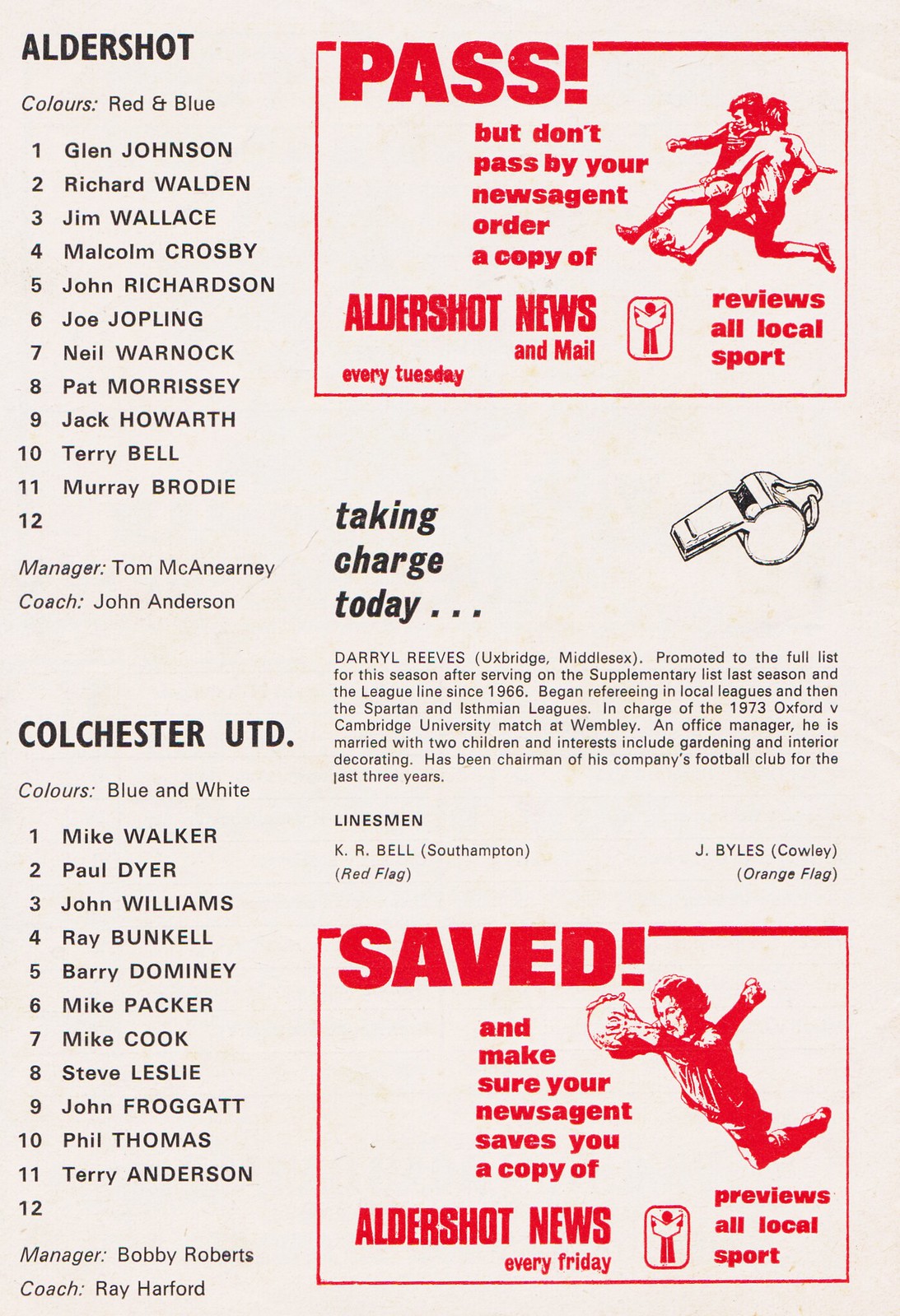The image is a vertically aligned rectangular snippet from a soccer program detailing a match between Aldershot and Colchester United. In the upper left corner, "Aldershot" is prominently displayed in bold, black, all-caps letters, followed by their colors, red and blue. Below this, there's a numerical list from 1 to 12 of the team's players, though number 12 has no name listed. At the bottom of this list, Aldershot's manager, Tom McKearney, and coach, John Anderson, are mentioned. Below this, "Colchester UTD" is also presented in bold, with their colors listed as blue and white. Their numerical list from 1 to 12 similarly leaves number 12 unnamed, and lists the manager, Bobby Roberts, and coach, Ray Harford.

On the right side of the image, in the upper corner, a red rectangular area catches the eye with "PASS!" in bold, red letters, followed by the prompt, "But don't pass by your news agent. Order a copy of Aldershot News," accompanied by an image of two people kicking a soccer ball. In the midsection on the right, there is an outline of a whistle next to the phrase "Taking charge today," followed by a paragraph of information. 

At the bottom right, another red-outlined rectangular area contains the word "SAVED!" in all-caps red letters and features an image of a person in mid-air holding a soccer ball. Below this, it advises readers, "Make sure your news agent saves you a copy of Aldershot News," emphasizing its comprehensive coverage of local sports.